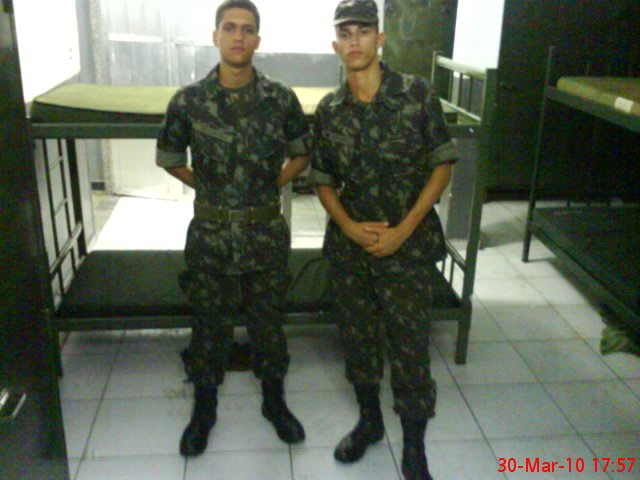This is a detailed photograph of two military personnel, possibly light-skinned and slightly darker-skinned, both standing in front of green metal bunk beds in what appears to be a barracks. The date in the bottom right corner of the image is marked in red letters as "30 MAR 2017 17:57." The floor consists of white square tiles, each approximately one foot per side, with black grouting in between. There is a diffused natural light coming through the windows in the background, creating a hazy atmosphere.

The soldier on the left is dressed in dark green camouflage uniform, including a top, bottom, and a green military belt cinched at the waist, with black boots completing the outfit. His hands are placed behind him. The soldier on the right, wearing a similar dark green camouflage uniform, has a dark baseball-style military cap and his hands are folded across his midriff. The green bunk beds behind them appear to have no bedding, just mattresses. There are additional details such as a locker visible off to the left, and a doorway, indicated by the presence of light.